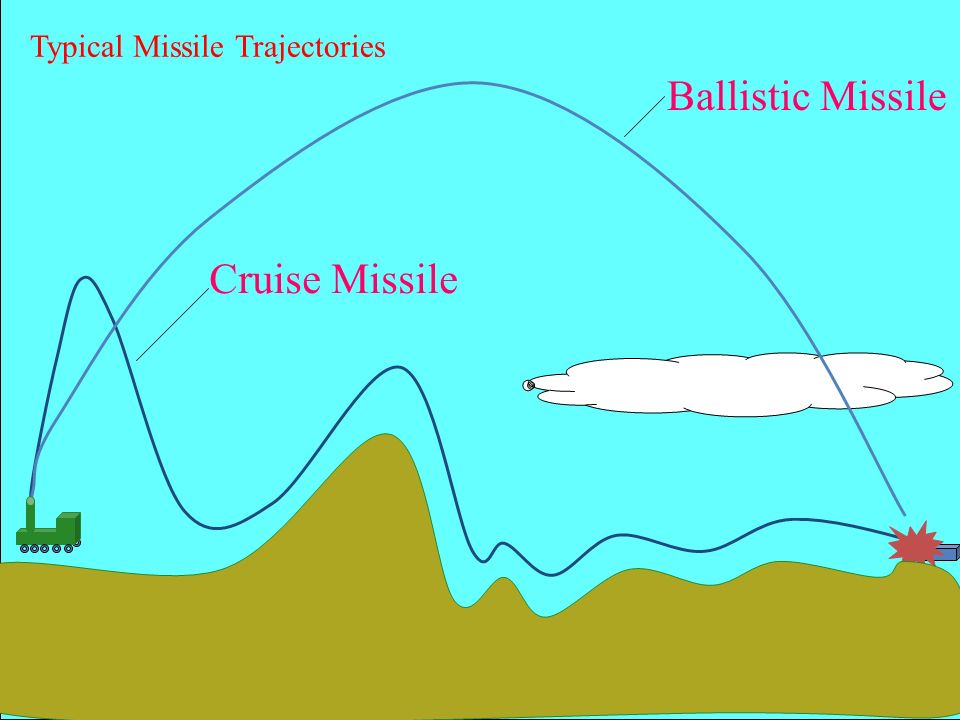The image illustrates typical missile trajectories against a solid light blue, sky-like background. In the upper left corner, purple letters spell out "Typical Missile Trajectories." A large arch labeled "Ballistic Missile" in a pink font dominates the view, stretching from the lower right, rising to the top middle, and descending to the lower left corner. Towards the bottom, an olive-green curved line, labeled "Cruise Missile" in pink, starts flat on the left, peaks, dips, and forms smaller waves as it extends rightward. At the base of the ballistic missile arch, a cartoonish green train with wheels is visible; above it, a squiggly line meanders up and down before settling into smaller undulations to the right. An elongated white cloud cuts across part of the arch on the right side. The image's lower section, primarily in olive green, has a truck-like figure near the left end of the ballistic missile trajectory and a red starburst towards the right.